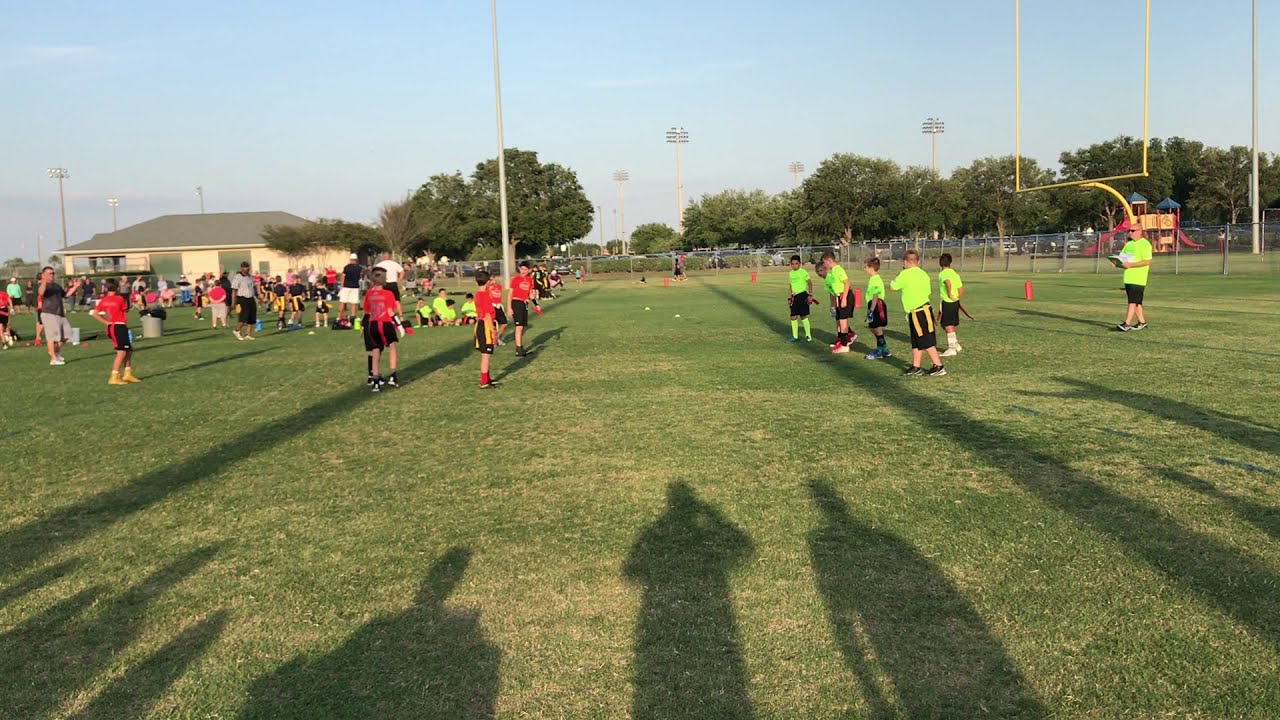The image captures a vibrant outdoor sports scene featuring a flag football game taking place on a football field with vividly green and yellow grass. In the foreground, shadows of spectators and possibly the photographer can be seen, suggesting a sunny day with the sun positioned behind them. The teams are distinguishable by their uniforms: the team on the left wears red T-shirts and black shorts, while the team on the right is in neon green T-shirts and black shorts. The coaches, dressed similarly to the players, are actively engaged with the kids.

In the background, there are various elements highlighting the lively environment. You can spot two adult men, likely coaches or parents, involved in guiding the children. Other children and parents watch the game from the sidelines. Further back, there are multiple ongoing games, with a soccer match also visible. The scene includes a yellow goal post, indicative of the football setting, and a chain-link fence along with a building on the left side, described as yellow with a gray roof. To the right, trees and a playground add to the picturesque landscape under a clear, blue sky. The image also shows lighting poles around the field and what appears to be a spectator area.